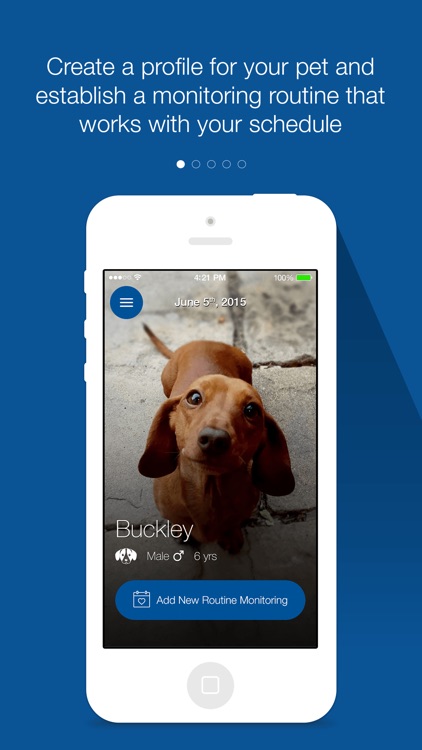Caption for Image: 
"Capture your pet's daily activity with our easy-to-use monitoring app! Featured in the digital display, Buckley, a healthy 6-year-old male Basset Hound with a sleek brown coat and long floppy ears, stands poised on a cement surface. The tail-wagging Buckley is visibly content as he gazes into the camera. Dated June 5th, 2015, at 4:21 PM, the app offers a seamless way to create a profile and establish a monitoring routine that aligns with your schedule. Simply tap the 'Add New Routine' button, adorned with a small white heart, to begin tracking your furry friend's well-being."